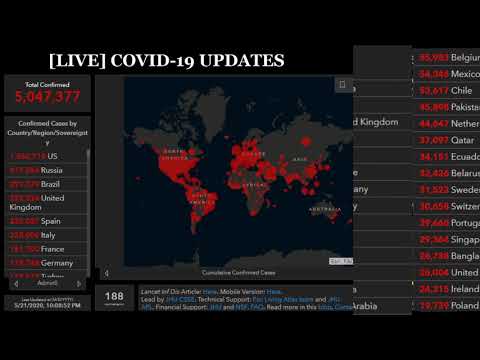The image appears to be a screengrab, likely from a website or broadcast, featuring live COVID-19 updates. The design includes black borders on the top and bottom, while the overall background is dark, utilizing shades of black, white, gray, and blue. At the top-left corner, white block letters spell out "Live: [COVID-19 Updates]." Central to the image is a dark-colored world map depicting all continents—North America, South America, Europe, Africa, Asia, and Australia. This map showcases several red hotspots, indicating areas with the highest concentration of COVID-19 cases, notably in North America, South America, Western Europe, and parts of Western Asia. 

On the left side of the image sits a column headed "Total Confirmed," which possibly lists cumulative case counts. Below this header, it states "Confirmed Cases by Country/Region," listing countries with significant case numbers such as the US, Russia, Brazil, UK, Spain, Italy, France, and Germany. The right side of the screen also features a country list including Belgium, Mexico, Chile, Pakistan, and the Netherlands, accompanied by numerical values, presumably representing confirmed cases. At the bottom, there is text likely referring to the medical personnel or entities responsible for updating the data. The overall imagery and data presentation suggest it was captured early during the COVID-19 pandemic.